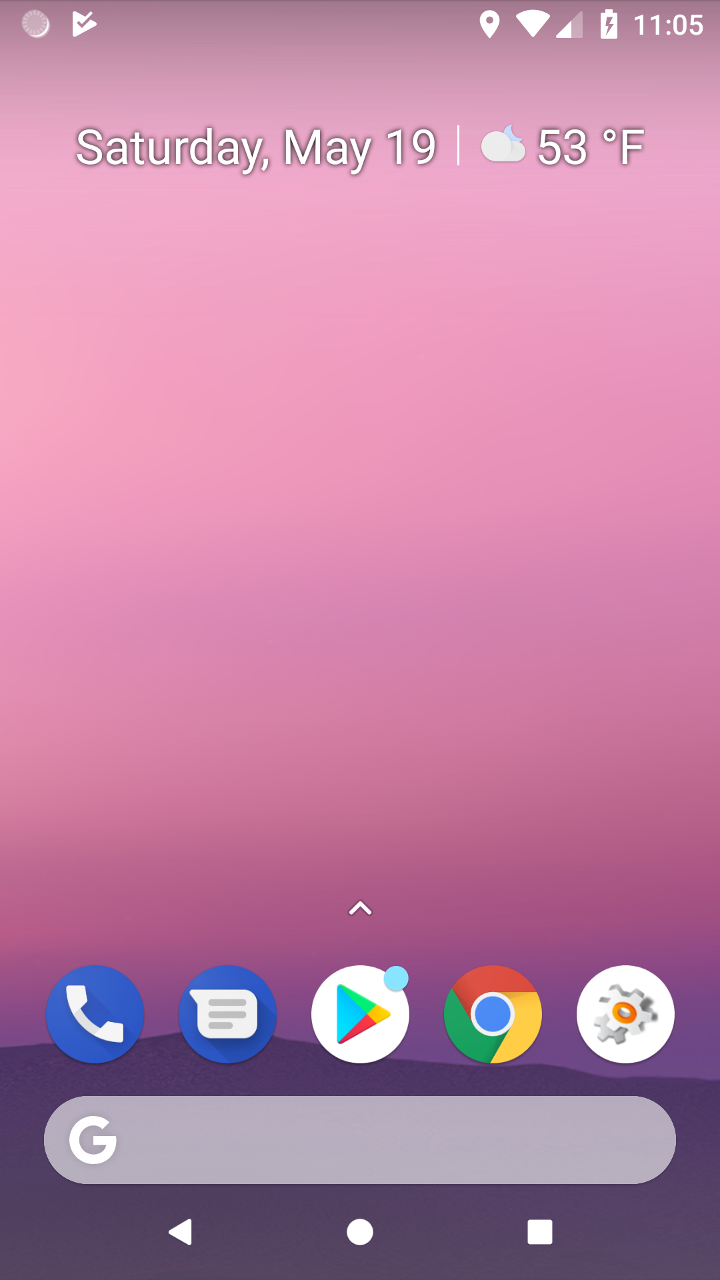This image showcases the home screen interface of a Google Pixel device, identifiable by its distinct software layout and navigation buttons. At the top of the screen, notifications are present alongside a to-do list checkmark icon. In the top right corner, there are icons for Google Maps, Wi-Fi with four bars, and cell signal strength showing half bars. The battery icon indicates a full charge at 100%, and the time displayed is 11:05. Directly below the time, the date reads Saturday, May 19th, and to the right, a weather icon featuring a cloud and moon shows the temperature as 53°F.

The background features a purple gradient, brightening towards the top and fading to darker hues at the bottom, with a scenic mountainscape subtly visible. The dock at the bottom of the screen contains icons for essential apps: Phone, Messages, Google Play Store, Chrome, and Settings. An upward arrow above the Google Play Store icon suggests that tapping it will reveal more applications.

Above this dock, a Google search bar is prominently displayed, marked by the Google "G" logo on the left and a text input field. Directly beneath the search bar, the device's navigation buttons include a back arrow, a circular home button, and a square for multitasking view.